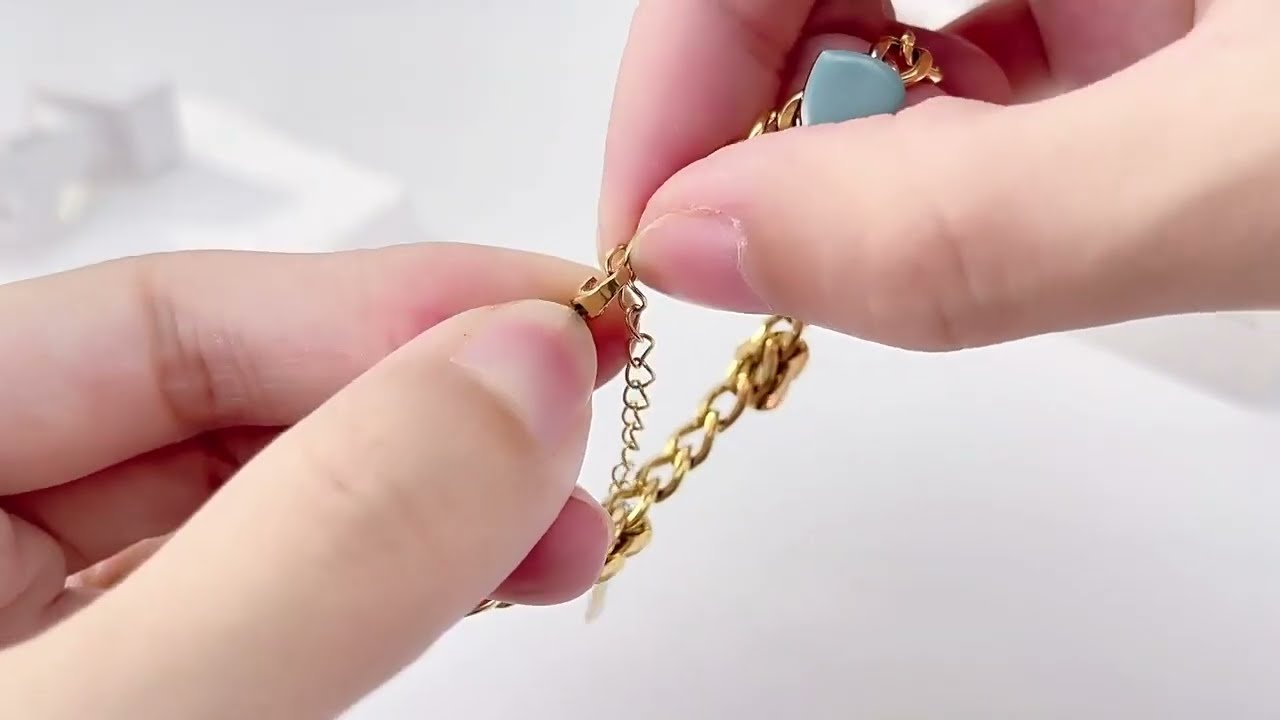In this wide rectangular photograph, a pair of hands with very light, Caucasian skin is delicately handling a golden chain against a stark white background. The image reveals the fingers, thumbs, and clipped nails of both hands without showing their palms. The left and right hands come from the lower left and upper right corners of the image, respectively. The gold chain is grasped between the thumbs and index fingers of both hands, with the clasp held prominently between them. 

The chain dangles towards the left hand before looping back up diagonally to the right hand, where a turquoise-colored trinket, possibly an upside-down heart pendant, is visible. The gold chain can also be seen wrapped around a finger on the right hand. A subtle shadow cast by the right hand appears on the white surface below, adding depth to the entirely white ground, which is accented by a set of white boxes with a yellow circle in the upper left corner. The hands exhibit a well-kept manicure, with nails clipped short and slightly curved, one nail on the left thumb showing a faint tint of pink.